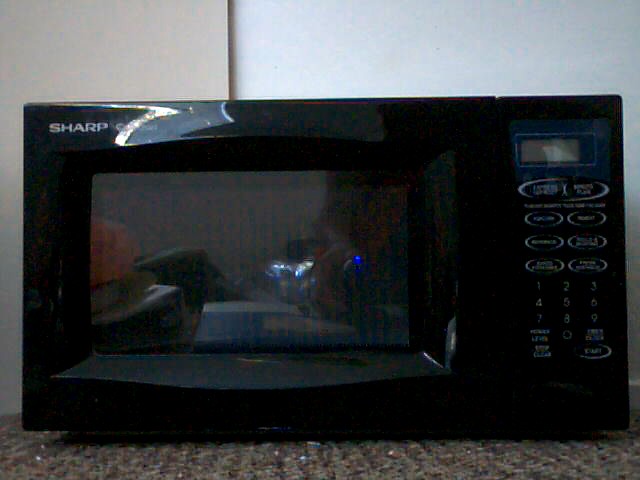The image is a rectangular photograph of a black Sharp microwave. The Sharp logo is positioned in white capital letters on the top left corner of the microwave's front. The microwave sits on an unsmooth, light brown surface that resembles the texture of wicker. The background features a wall with a light tan section on the left and the rest appearing white.

The front of the microwave has a reflective glass door, revealing a vague reflection of items and possibly the photographer. The right-hand side of the microwave has a gray display bordered in white. Below the display, there are oval buttons arranged from top to middle, each representing different functions. Beneath these, a numeric keypad displays numbers 1 to 9 in a left-to-right sequence, with a 0 in the center and additional unlabeled buttons on the right-hand side. Despite some of the functions and buttons being unreadable due to glare and graininess, the photo shows the general layout typical of microwaves, including buttons for defrosting and cooking. The photo itself is grainy, adding to the difficulty in discerning finer details. Behind the microwave is a simple white drywall.